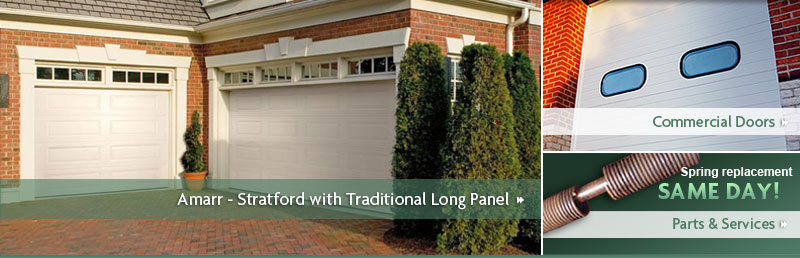The image showcases three distinct banners, each highlighting different aspects of garage doors and related services:

1. The first banner prominently features a red brick house with two white garage doors. The banner placed over these doors reads "Omar - Stratford with Traditional Long Panel," accompanied by a forward arrow. The setting includes a red brick driveway and some greenery flanking the sides of the garage doors, enhancing the residential ambiance.

2. The second banner, located in the top right corner, provides a closer view of one of the garage doors. This door is marked by a banner that says "Commercial Doors." The door itself is a white panel design with two windows placed in the middle, resembling a pair of eyes.

3. The third banner, situated in the bottom right corner, displays a brown object against a dark green background. The text on this banner advertises "Same Day Parts and Services" and highlights the company's commitment to offering swift replacements.

Each banner serves to illustrate different aspects of garage door styles and services available.